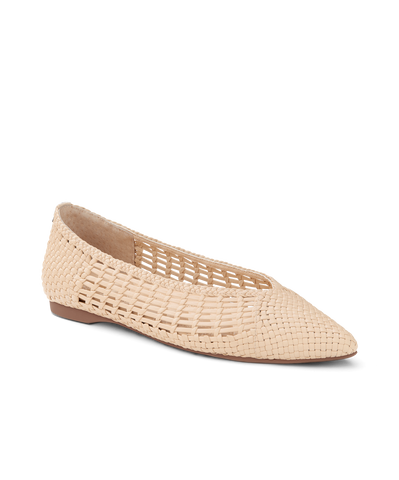This product photo showcases a single women's ballerina flat shoe set against a completely white background. The shoe boasts a distinct basket weave pattern, intricately crafted from what appears to be leather or a similar fabric. Its light, cream-colored canvas gives it a slightly darker than typical beige tone. The design features a pointed toe area with a tightly woven texture, transitioning to a larger, more breathable weave along the sides, and tightening again towards the back. The shoe has a very short heel, approximately half an inch, in dark brown, possibly wooden. The interior by the heel is lined with leather, adding a touch of elegance to this simple yet stylish flat.